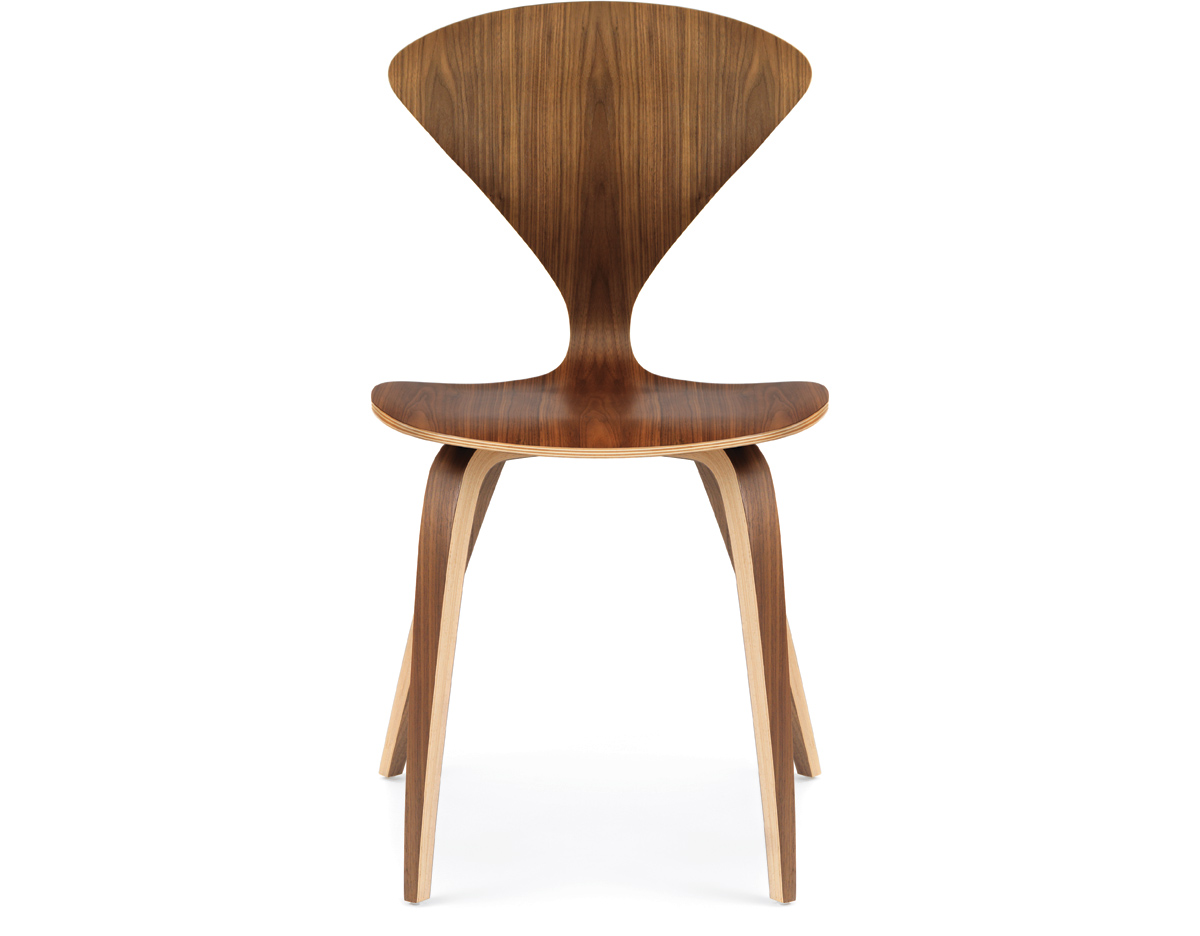This image, in portrait orientation, features a modern Art Deco-style chair prominently displayed against a primarily white background that transitions to a lighter gray at the bottom. The chair, crafted from dark walnut wood, showcases a visually striking hourglass design where the back and seat are both fan-shaped, curving to connect at a narrow section in the middle. The seat is a regular size, while the back, despite being slender in the middle, widens towards the top for a unique aesthetic. The legs, framed in a lighter, almost white wood, slightly curve outward, providing a sturdy base. This photograph emphasizes the chair's elegant, grainy wood texture and minimalist design, appearing to float on the stark white background typical of product photography.